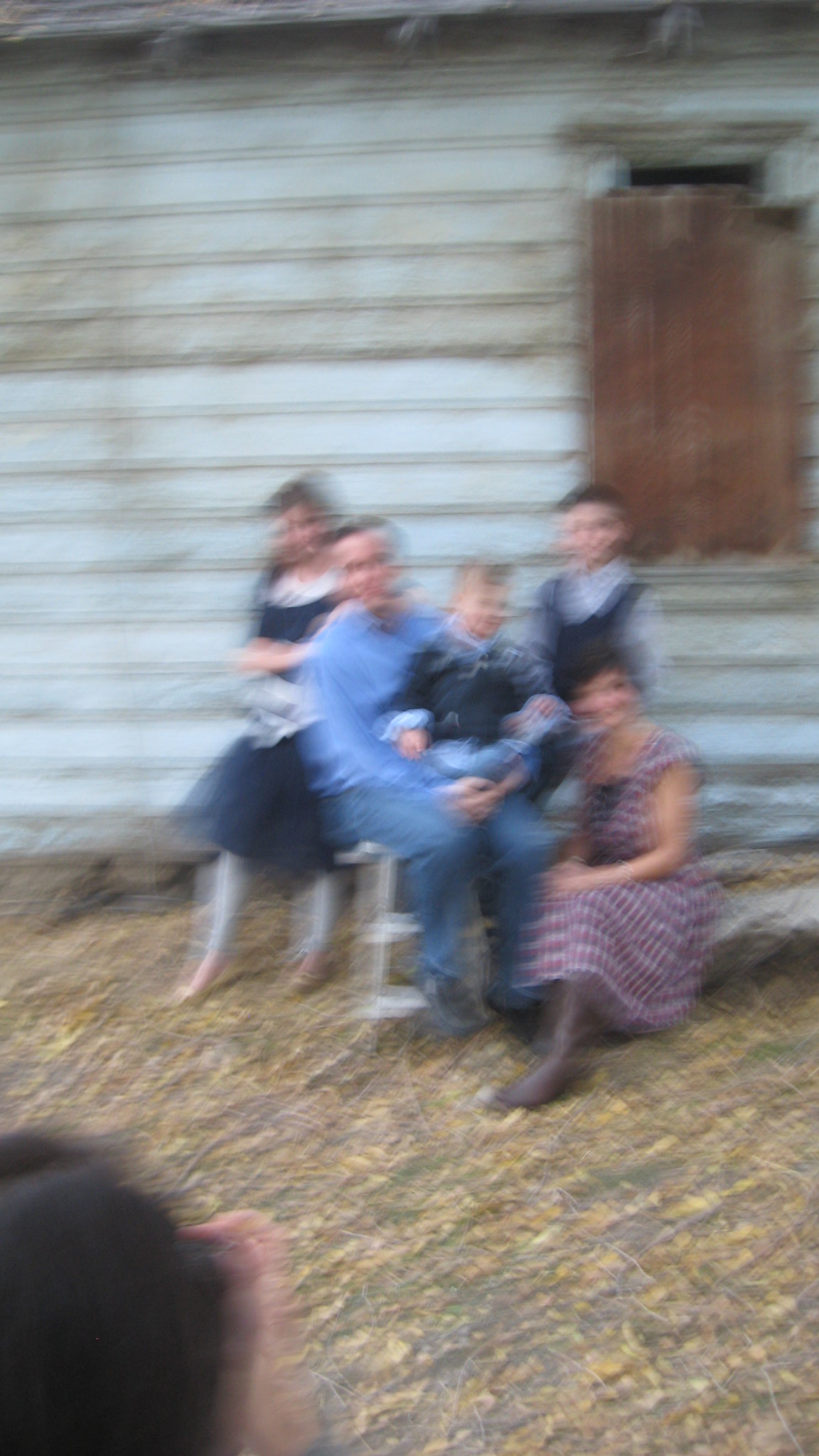This is a family photograph taken outside of a house in what appears to be a rural area on an overcast day, contributing to a darker, motion-blurred image. The central figure is a man seated on a white chair, wearing a long-sleeved blue shirt and jeans. He holds a small child clad in a blue vest over a light blue shirt. To the man's right stands another young boy, also in a blue vest and a long-sleeved shirt, next to a woman kneeling in a red and white plaid dress, brown cowboy boots, and a silver bracelet on her arm. The woman has short hair and appears to be smiling. Beside her, a girl in a black dress with white lace around the midsection stands with her arms crossed, wearing white shoes. The background is marked by a house with boarded-up windows and fall leaves scattered on the ground. The photograph inadvertently includes the head and right hand of the person taking the picture in the bottom left-hand corner.